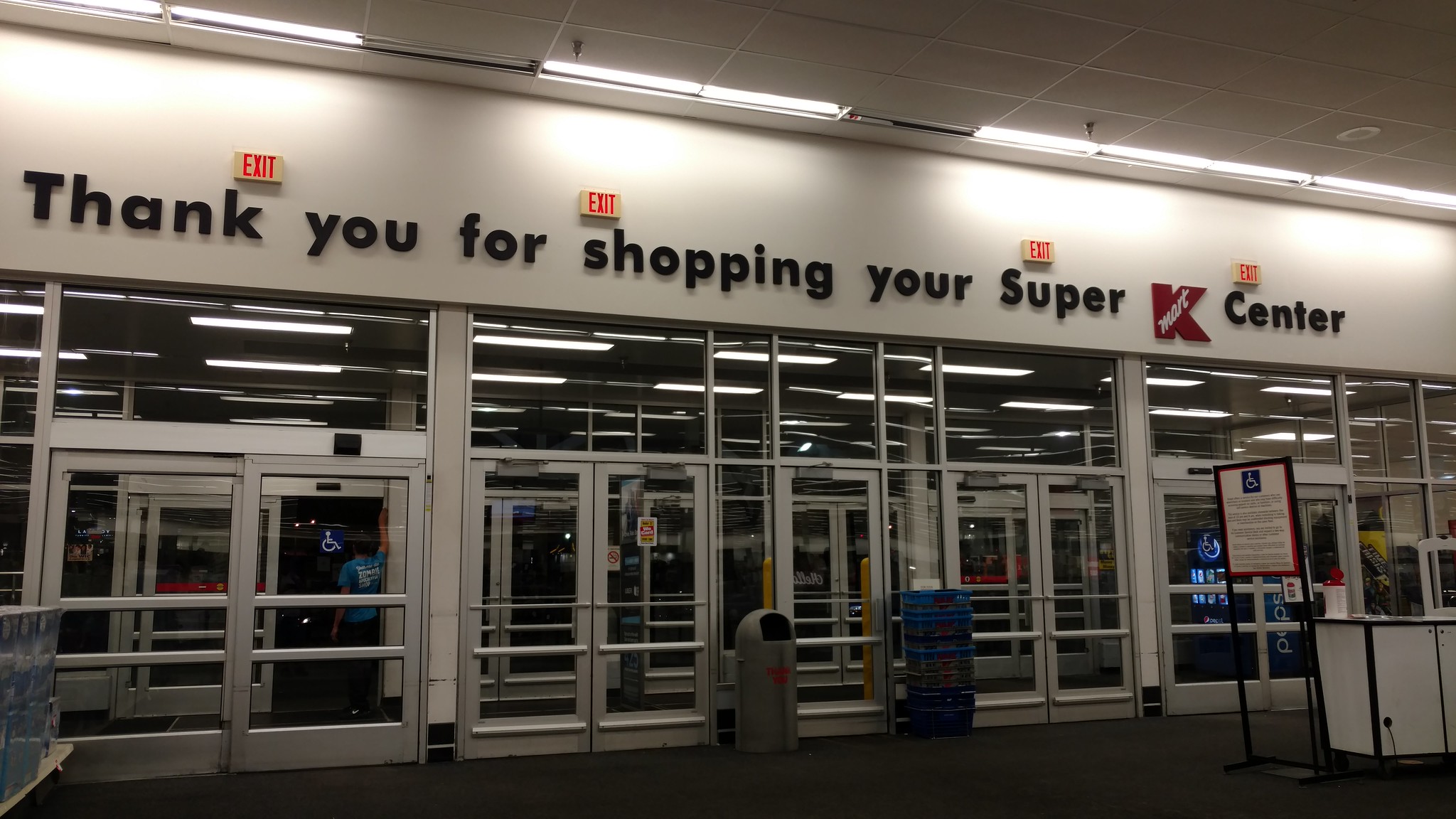This interior photograph of a now-defunct Kmart captures the exit area with meticulous detail. Above the glass doors, the drop ceiling features standard ceiling tiles interspersed with LED lights. The white section of the wall above the doors prominently displays the message "Thank you for shopping your Super K Center" in black lettering. Positioned above this text are four exit signs. The exit area includes three sets of doors: automatic double doors on both the left and right sides and five manual push doors in the center. A man in a blue shirt is seen walking out through the automatic doors on the left. In front of the center push doors, there is a neatly stacked pile of ten to fifteen blue carry baskets next to a gray garbage can. The store's gray carpet leads to a small white desk that holds a sign, presumably indicating handicap accessibility.